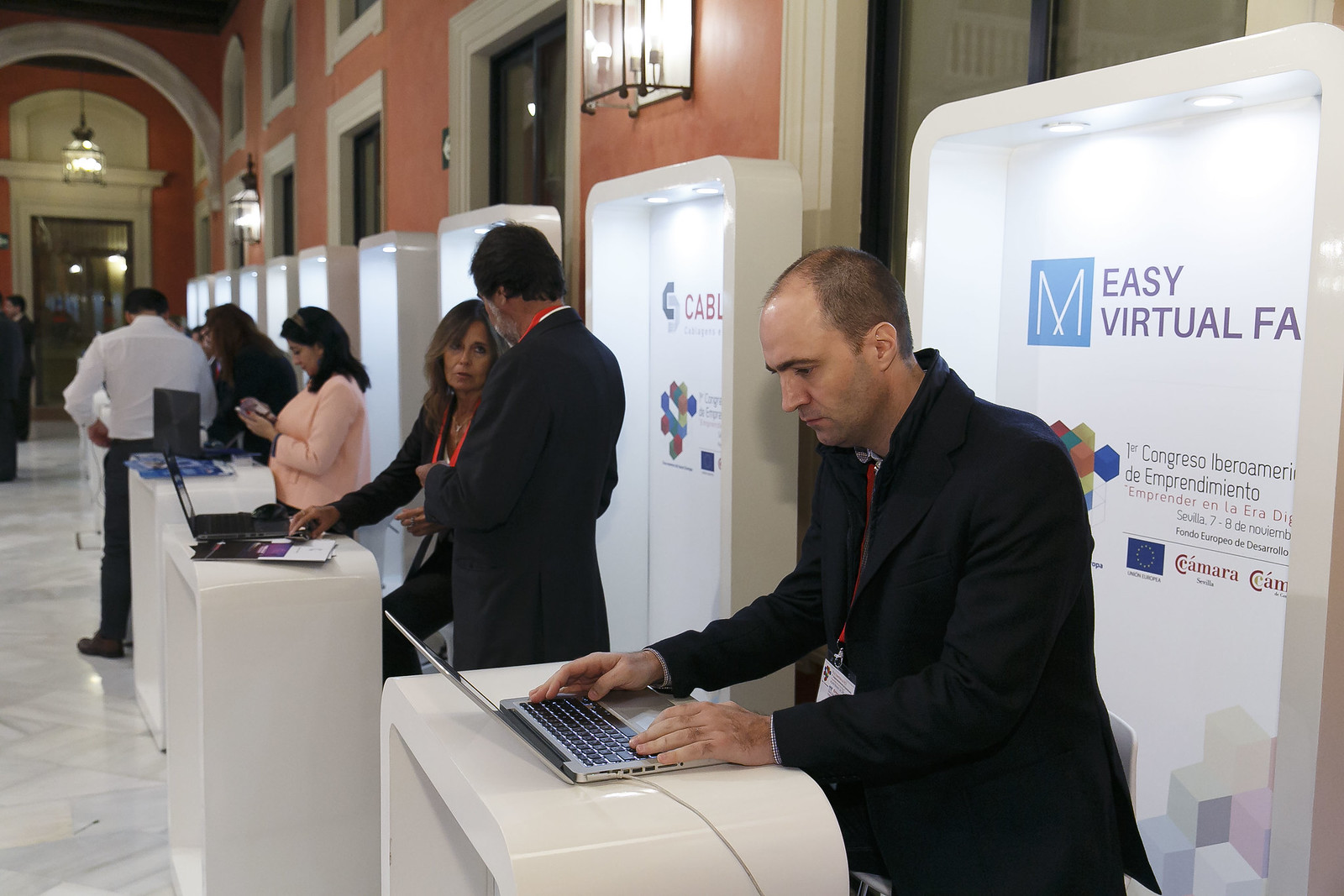In this photograph, a line of individuals is seen positioned diagonally at what appears to be a conference event. They are engaging with their laptops on white, lectern-shaped desks, each accompanied by a rectangular white-framed sign behind them—these signs display various texts related to the conference.

At the forefront is a man in a black suit with a red lanyard around his neck, intently working on his silver laptop, which is plugged in. The prominent sign behind him reads "EZ Virtual FA" with additional Spanish text, "Congreso Iberoamerica de Emprendimiento Emprender en la Era Digital." His commitment is evident as both hands rest on the keyboard. 

To his side, proceeding along the line, are additional participants. Directly next to him stands a man and a woman in conversation, while further down, a woman dressed in a peach top concentrates on her device. At the far end, another pair—a man and a woman—are engaged in their tasks. 

The setting features a white marble floor, adding to the sleek, professional ambiance of the event. The collective attire of the individuals spans a range from light colors like pink and peach to darker shades, emphasizing the formality and diversity of the occasion. This image captures a moment of focused activity and professional interaction at what is likely a tech-centric conference.